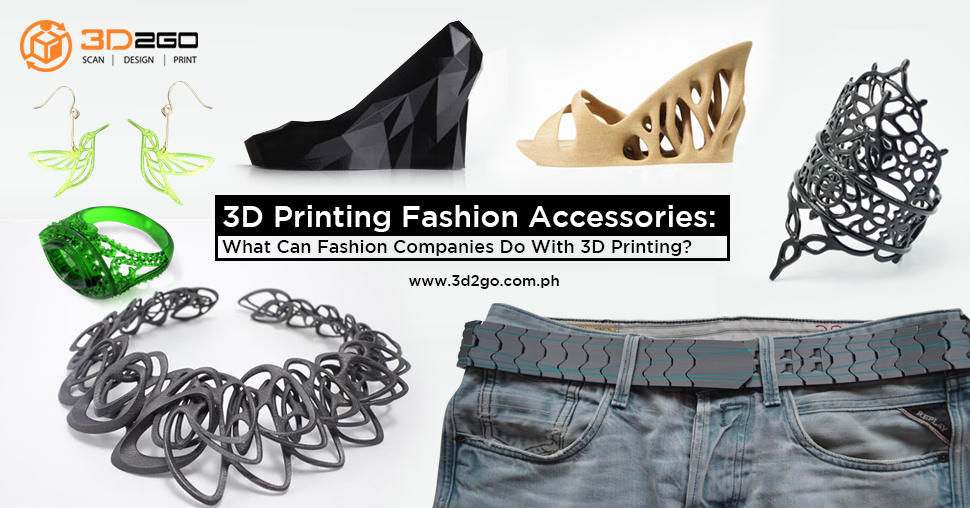This captivating image showcases the innovative realm of 3D printed fashion accessories, illustrated with a vivid assortment of items. Featured prominently are green hummingbird earrings, green rings, a dark silver necklace, and a dark silver bracelet. The image exhibits a mix of footwear including black high heels, a black geometric wedge, and a beige sandal reminiscent of Yeezy designs. Additionally, it presents blue jeans paired with a black iron belt. The scene is marked by vibrant colors with green accessories, blue jeans, and contrasting black and beige footwear. In the top left corner, the logo of 3D2Go – Scan, Design, Print – is displayed, enhancing the brand's identity. The logo is characterized by an orange cube with arrows pointing in various directions. Centrally positioned text poses the question, "What can fashion companies do with 3D printing?" and provides a direct link to their website, www.3d2go.com.ph, inviting viewers to explore further.